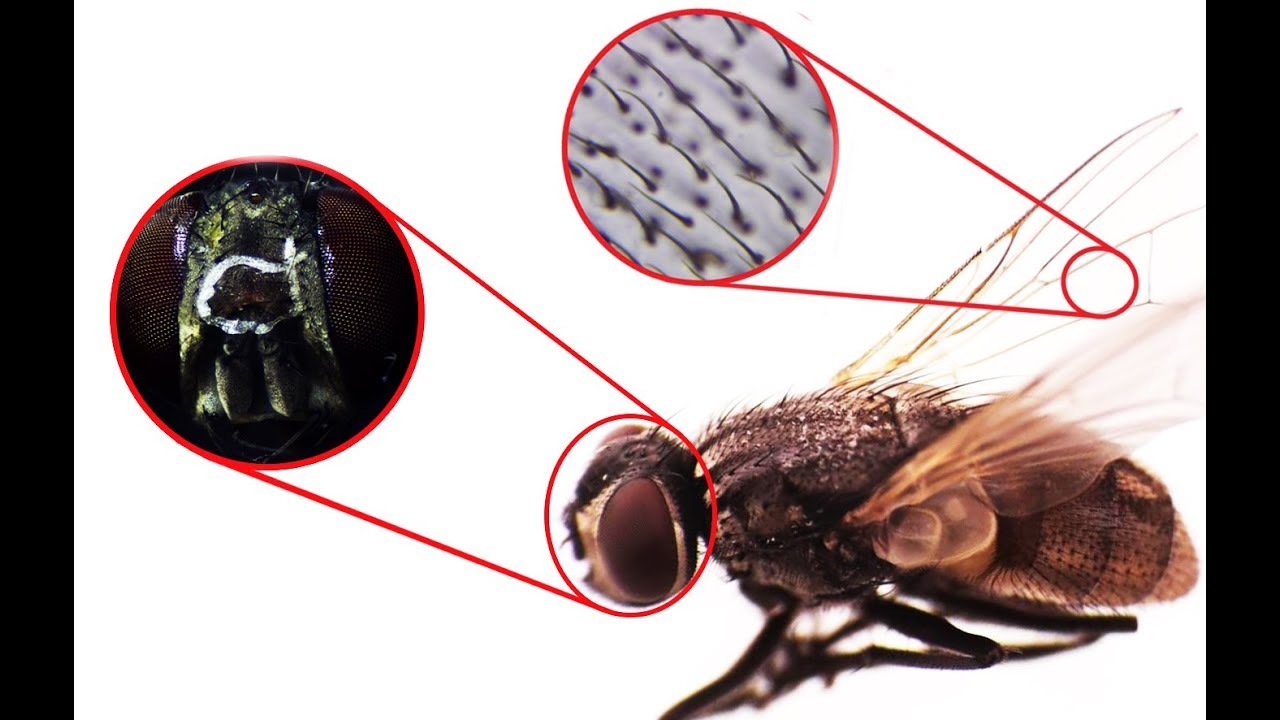The image is an informational graphic, possibly a still frame from a video, featuring a detailed depiction of a fly. The fly is positioned in the bottom right quadrant against a white background, enclosed by black vertical bars on the left and right sides. The fly's body is compact, mostly brown with a beige hue towards the end, and it has long, semi-transparent wings through which the body is partially visible. Its most striking feature is the pair of large, dark reddish-burgundy eyes. Overlaying the fly are smaller circles with zoomed-in views connected by lines. One circle highlights the intricate, segmented structure of the fly's eyes, while another focuses on the tiny hairs on the wings. The graphic emphasizes these details to illustrate the fly's anatomy closely.